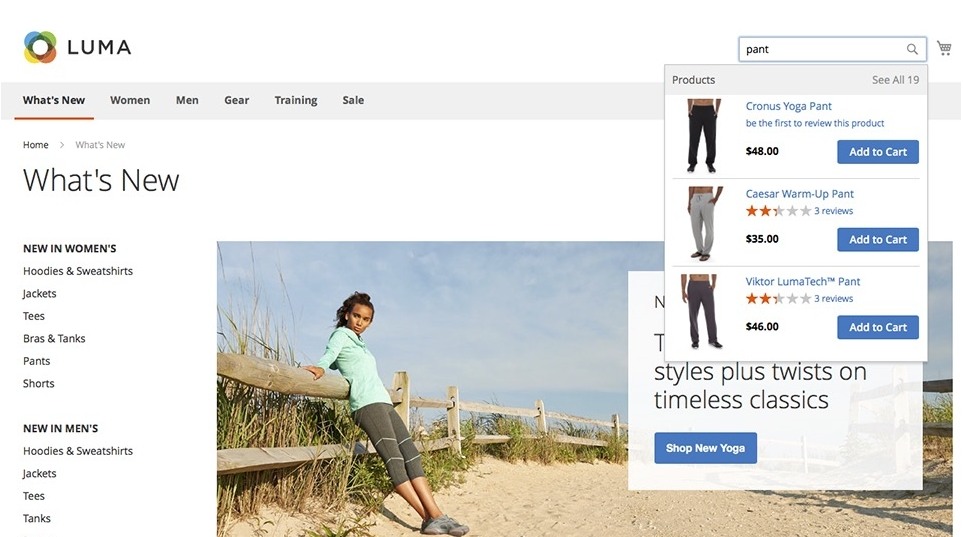The image features a cropped section of a webpage belonging to a website named "Luma," as indicated by the black-lettered logo on the top left. Adjacent to the logo, there's a search bar with the word "Pant" typed in, accompanied by a shopping cart icon embedded within the search bar. Beneath the search bar, a pop-up box appears with a grey header labeled "Products" on the left and "See all 19" on the right. This box contains three listings for different types of pants, each illustrated with a thumbnail on the left and accompanied by descriptions, prices, and ratings on the right. Each listing also includes an "Add to Cart" button at the bottom right corner.

Above the search bar, there is a horizontal grey navigation bar featuring categories such as "What's New," "Women," "Men," "Gear," "Training," and "Sale." The "What's New" category is currently highlighted with an orange horizontal bar beneath it. Below this navigation bar, the webpage transitions into the main body with a white background. 

At the top-left corner of this section, breadcrumb text reads "Home" and "What's New," leading into a prominent header that states "What's New" in large black letters. The right side of the page showcases a large photograph of a woman leaning against a fence along a sandy walkway. To the right of the image, the text "What's New in Women's" stands out in bold black letters, followed by several categories listed underneath. Further down, similar text indicates "What's New in Men's," which also has corresponding categories listed beneath it.